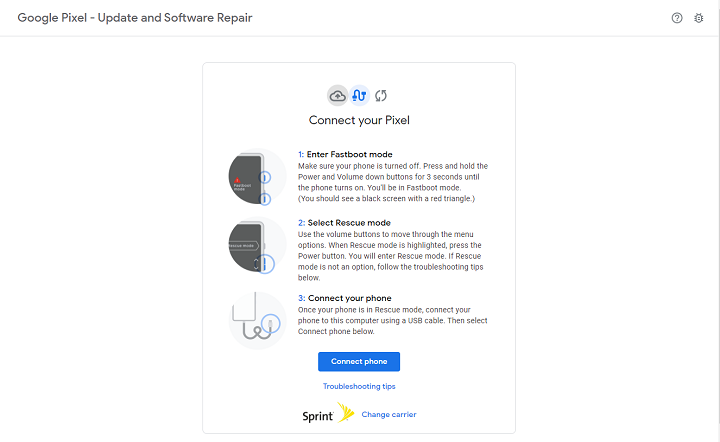In this informative image, the background is entirely white. At the top left corner, the text reads "Google Pixel Update and Software Repair." The top right corner features a circular icon containing a question mark, next to a message icon. Centrally located is a detailed instructional message box with various icons and text to guide the user through connecting their Google Pixel device.

**Main Instructions:**
1. **Connect Your Pixel:**
    - An icon of a cloud with connecting arrows forms a circular motion.
    - **Step 1:** "Enter Fast Boot Mode" – Accompanied by a paragraph explaining the procedure.
    - **Step 2:** "Select Rescue Mode" – Another paragraph provides detailed instructions.
    - **Step 3:** "Connect Your Phone" – Includes a paragraph with further details.

Illustrative icons next to each step visually demonstrate the process.

Toward the bottom, a bright blue label with white text instructs users to "Connect Phone." Beneath this label, there is another section with a white background featuring the text "Troubleshooting Tips" in blue.

Additionally, the black-colored Sprint logo with the word "Sprint" appears, accompanied by the option "Change Carrier" in blue text.

Overall, this image serves as a step-by-step visual guide for updating and repairing Google Pixel software, complete with icons to assist users through the process.